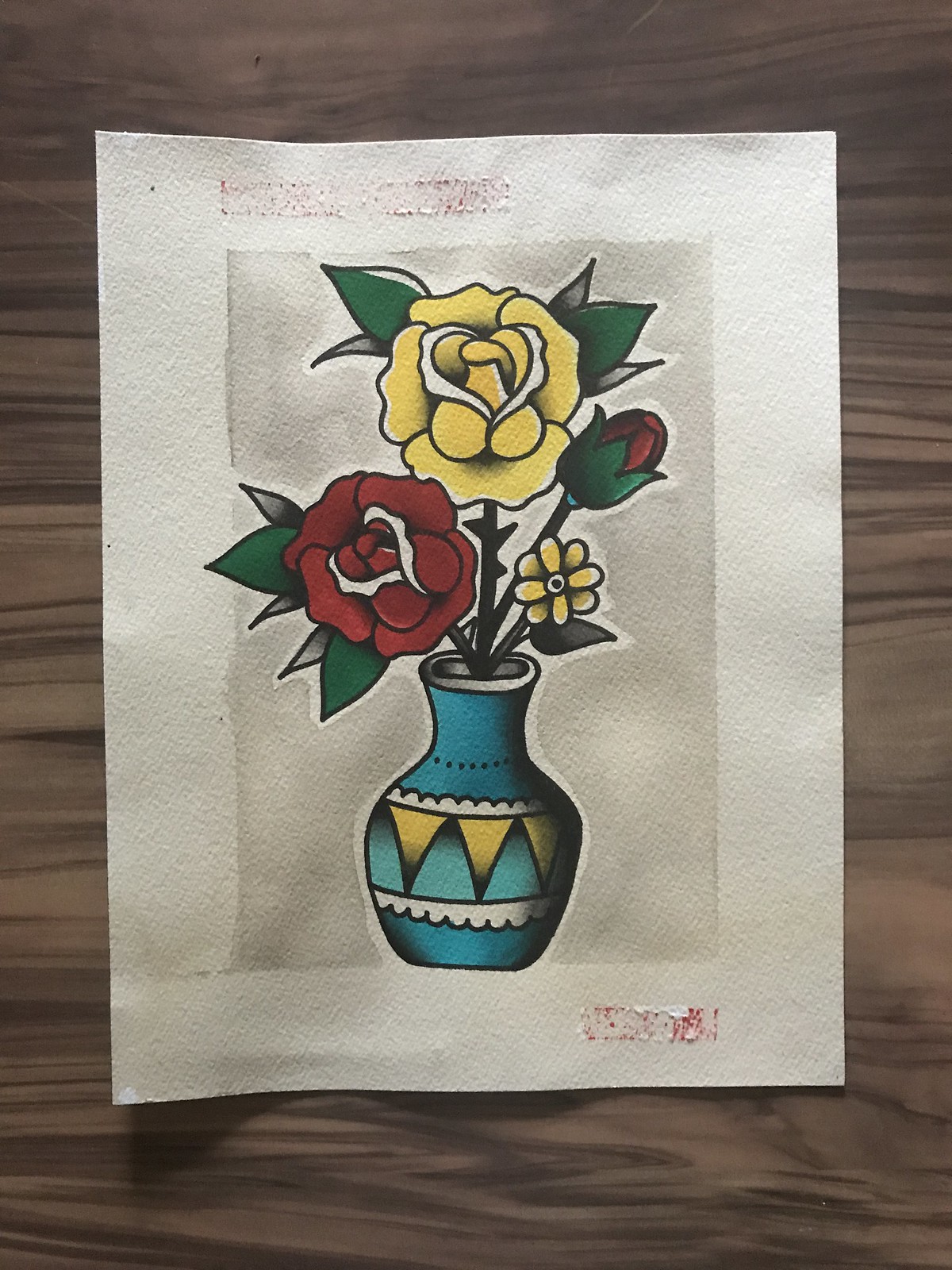The illustration is displayed on a piece of white matte paper, which is placed on a brown wooden surface characterized by its noticeable graining and wavy texture. Central to the illustration is a blue vase adorned with two white bubbly bands circling it. Separating these bands are three yellow triangles. Emerging from the vase are several flowers, notably including a red rose with two small white petals, a yellow rose with a similar pair of white petals, and a rosebud still surrounded by green foliage. Additionally, there is a yellow flower resembling a small daisy. Each rose is accompanied by vibrant green leaves, adding depth and contrast to the arrangement.